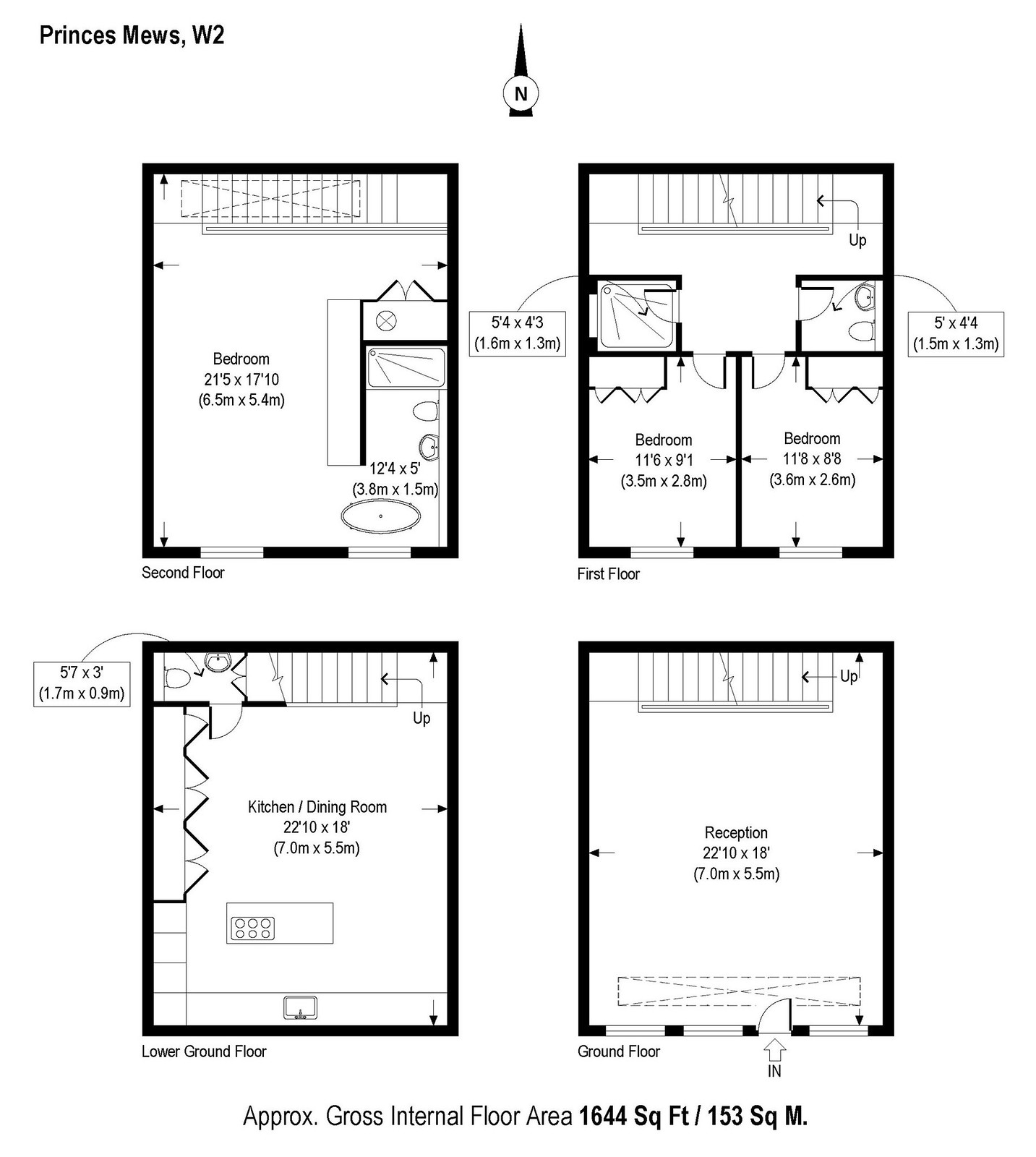This detailed photo showcases four floor plans, arranged in a grid with two on the top and two on the bottom, each spaced evenly. Starting from the top-left, the first floor plan features a single bedroom. Moving to the top-right, the second plan includes two bedrooms, each with its own adjacent bathroom, situated behind the bedrooms along with a staircase. Transitioning to the bottom row, the bottom-left floor plan is designated as a kitchen/dining room area, measuring 22 feet 10 inches by 18 feet, with the kitchen located along the back wall. The final plan on the bottom-right indicates a reception area, accompanied by a bathroom situated at the bottom-left corner, and another bathroom located at the top-right corner.